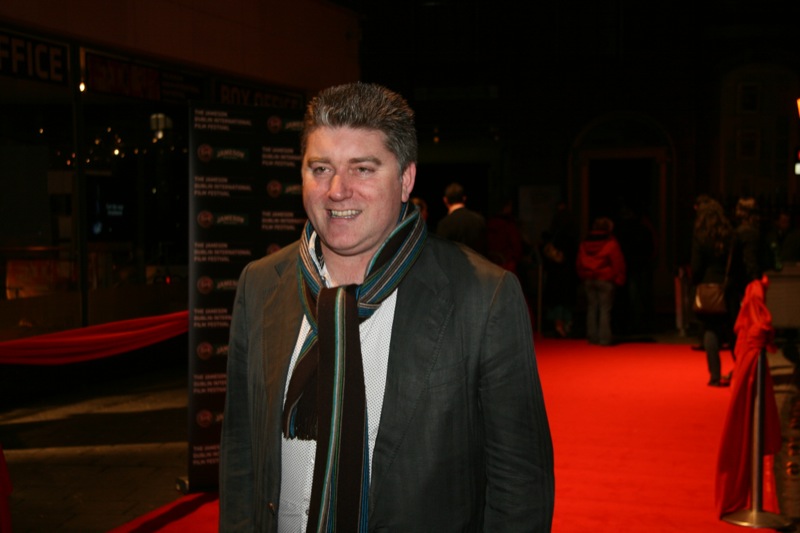In this detailed photograph, a man is standing on a stark red carpet inside a large, dimly lit room that resembles a theater. There are gold poles with wrapped red sheets creating elegant lines on the carpet. To his left, a mirror reflects some shadowy forms, adding depth to the scene. Behind him, rows of seats flank one side of the room, and several indistinct people mill about in the background, partially obscured by the low lighting. The man, smiling at the camera, is well-dressed in a casual brown blazer (which appears charcoal gray in some light) over a white shirt, accessorized with a striped scarf in shades of black, teal, and burgundy. His short, spiky brown hair, with a hint of gray, frames his full face. There’s an illegible large sign behind him, adding to the ambiance of this sophisticated setting. Additionally, a few steps lead up to another area on his right, further suggesting the grandeur of the space.